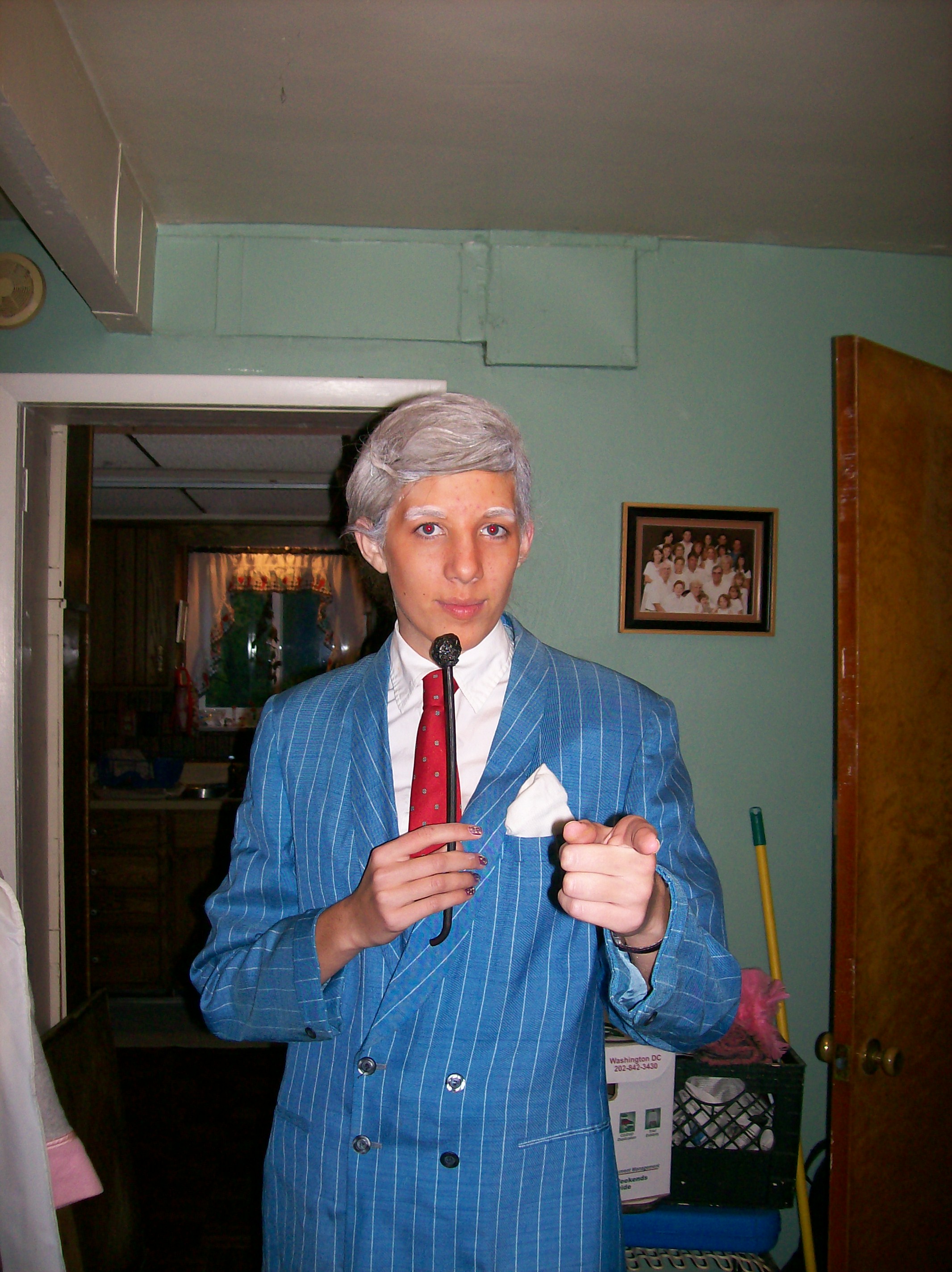The photograph captures a young man, possibly a teenager or in his early twenties, dressed in a detailed costume that evokes the appearance of a vintage television host, perhaps resembling Johnny Carson. He has tan brown skin and wears a short, voluminous grey wig with matching painted white eyebrows. Standing at the center of the image, he looks directly at the camera with one hand pointing towards it and the other holding a slender microphone with a round head, reminiscent of those used in the 1980s. His attire is a blue and white pinstriped suit jacket over a white button-up shirt, accessorized with a red tie featuring grey dots and a white handkerchief neatly tucked into his chest pocket.

The setting is an interior room with a white-painted ceiling and light green walls. To the right, there is an open, slightly worn light brown door with a bronze doorknob, leading to a shadowy area that might be another room or a bathroom. Further details in the background include a black and gold framed family photo hung on the green wall, a black crate, and a partially visible yellow broom handle. The overall lighting of the room is dim, adding a certain ambiance to the scene.